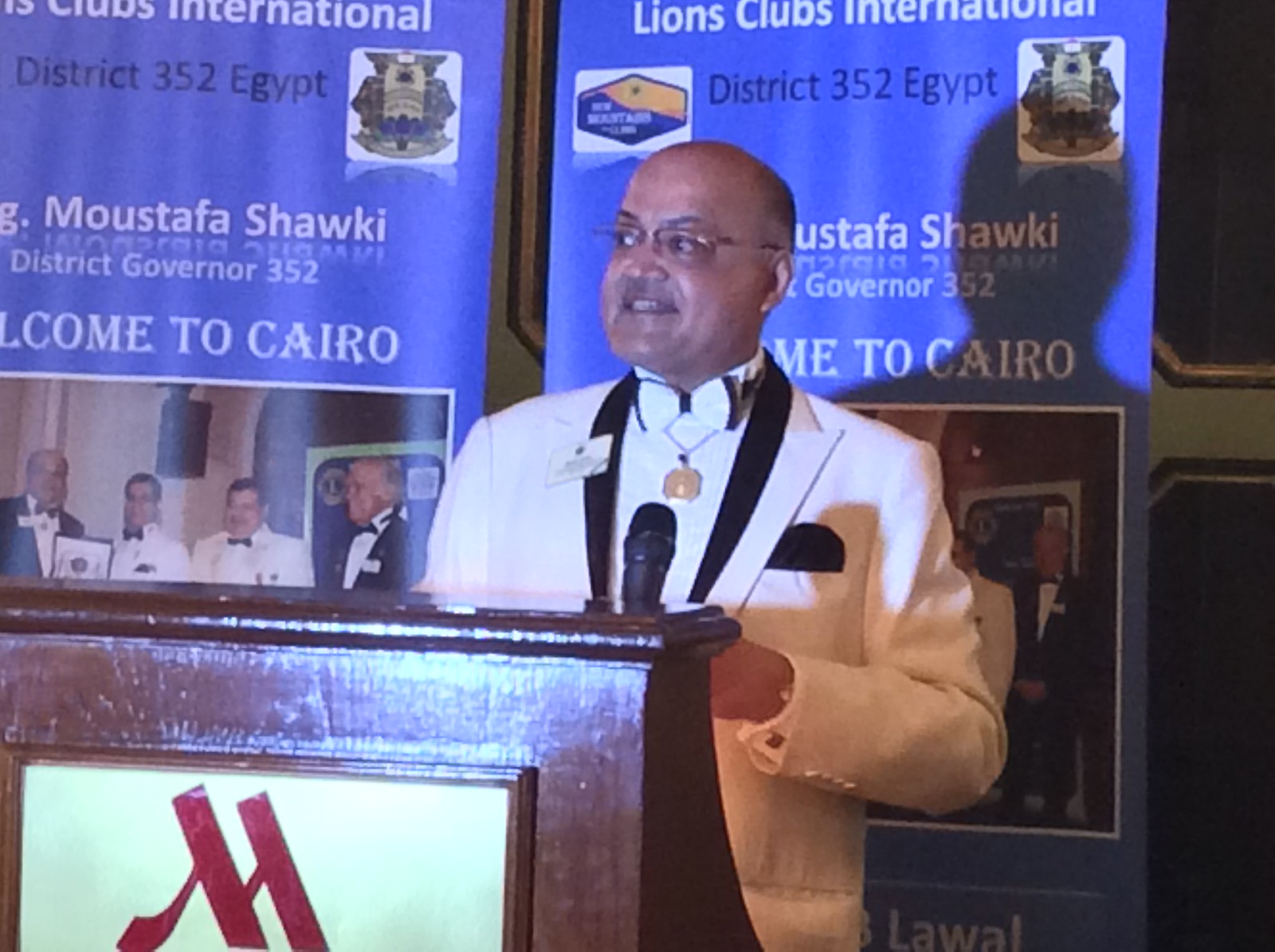In this photograph, an older gentleman with glasses and a bald head is speaking at a brown wooden podium featuring the Marriott logo. He is dressed in a distinctive white tuxedo jacket with black lapels, a white and black bow tie, a black vest, and a notable gold medal hanging around his neck. The name tag pinned to his left lapel adds to his formal appearance. The man is positioned in front of a blue backdrop adorned with white text and logos, which includes "Lions Club International, District 352 Egypt, Mustafa Schauke, District Governor 352, Welcome to Cairo." This context suggests he is addressing a Lions Club International conference or banquet. A bright spotlight illuminates him, casting a shadow on the backdrop, highlighting his presence at the event.